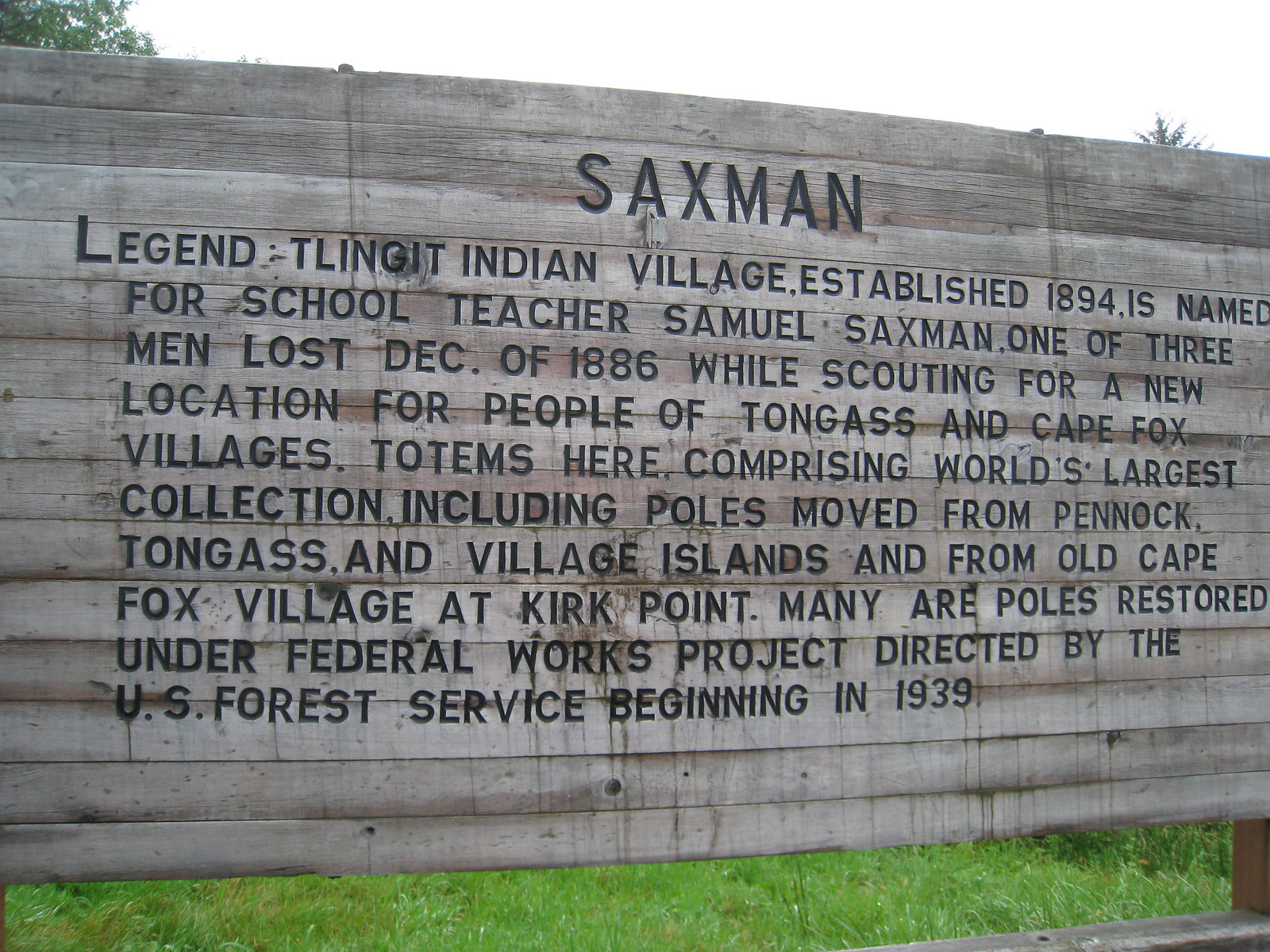The image depicts a wooden sign constructed from numerous stacked planks, situated outdoors in a field of green grass. Intricate carvings on the sign, highlighted in black paint, catch the eye and convey historical information. The top title reads "SAXMAN" in bold capital letters, followed by a detailed inscription: "Legend Tlingit Indian Village, established in 1894, is named for school teacher Samuel Saxman, one of three men lost in December of 1886 while scouting for a new location for the people of Tongass and Cape Fox Villages. Totems here comprise the world's largest collection, including poles moved from Pennock, Tongass, and Village Islands, as well as from Old Cape Fox Village at Kirk Point. Many of the poles were restored under a Federal Works Project directed by the U.S. Forest Service beginning in 1939." The sign, positioned with a small gap at the bottom revealing the grass behind it, appears slightly weathered with some text beginning to fade. Above it, the scene is framed by a white sky with treetops and leaves peeking in from the top left and top right corners. In the bottom right, a glimpse of a fence with a railing is visible.